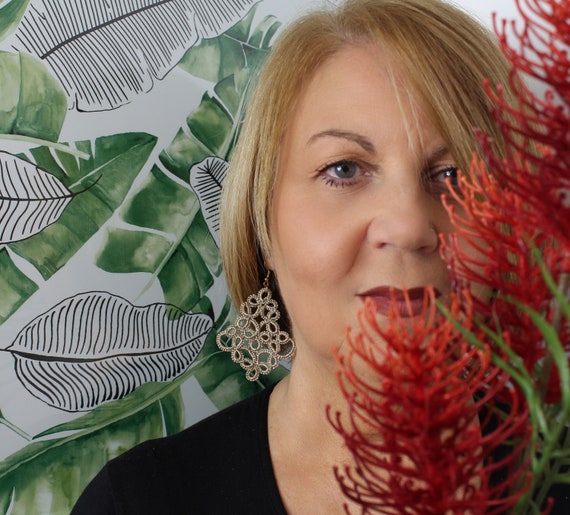The image is a detailed close-up portrait of a middle-aged Caucasian woman with short to medium blonde hair, wearing noticeable makeup including mascara and dark red lipstick. She is adorned with a long dangling earring designed with intricate flower-like or lacy, curly-Q patterns. The woman is partly obscured by a reddish-orange, almost plastic-looking plant that resembles algae or an Australian bottle brush, with thin layers extending outward, giving an under-the-sea or fishbowl ambiance. She is dressed in a black scoop neck top, visible from her upper chest to the top of her head. The background features a fabric or wallpaper with a tropical motif, displaying large green leaves and smaller leaves outlined in black and white. The woman has greenish-blue eyes and presents a subtle half-smile.